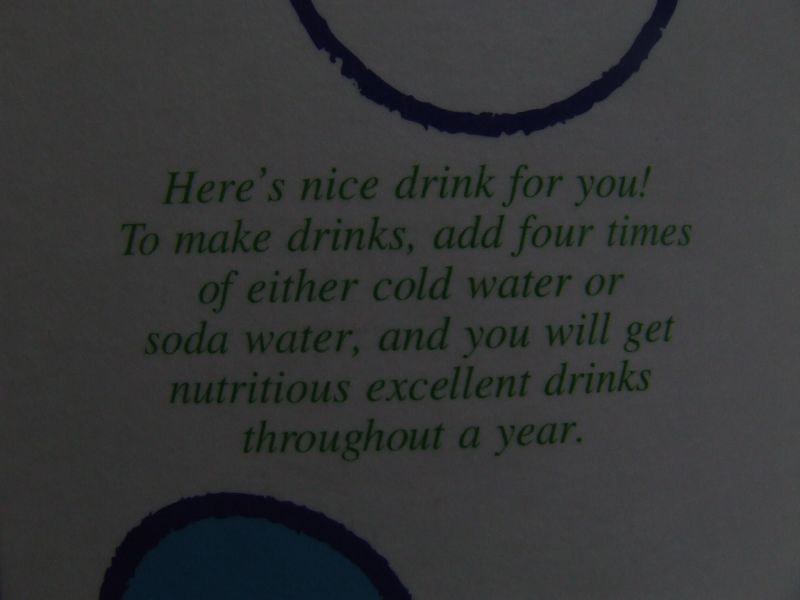The image features a white page with slightly fuzzy texture, bearing a central message in green text that reads: "Here's nice drink for you! To make drinks, add four times of either cold water or soda water, and you will get nutritious, excellent drinks throughout a year." The page is devoid of any artist copyright or additional text.

At the top of the page is a white circle outlined in black, positioned slightly off-center to the right. Similarly, at the bottom left, there's a navy blue or black-outlined circle that is filled with a pretty blue shade but is partially cut off. The overall background of the image appears to be a light to medium gray. The font of the text is dark green and slightly slanted, and the language used suggests it is not native English.